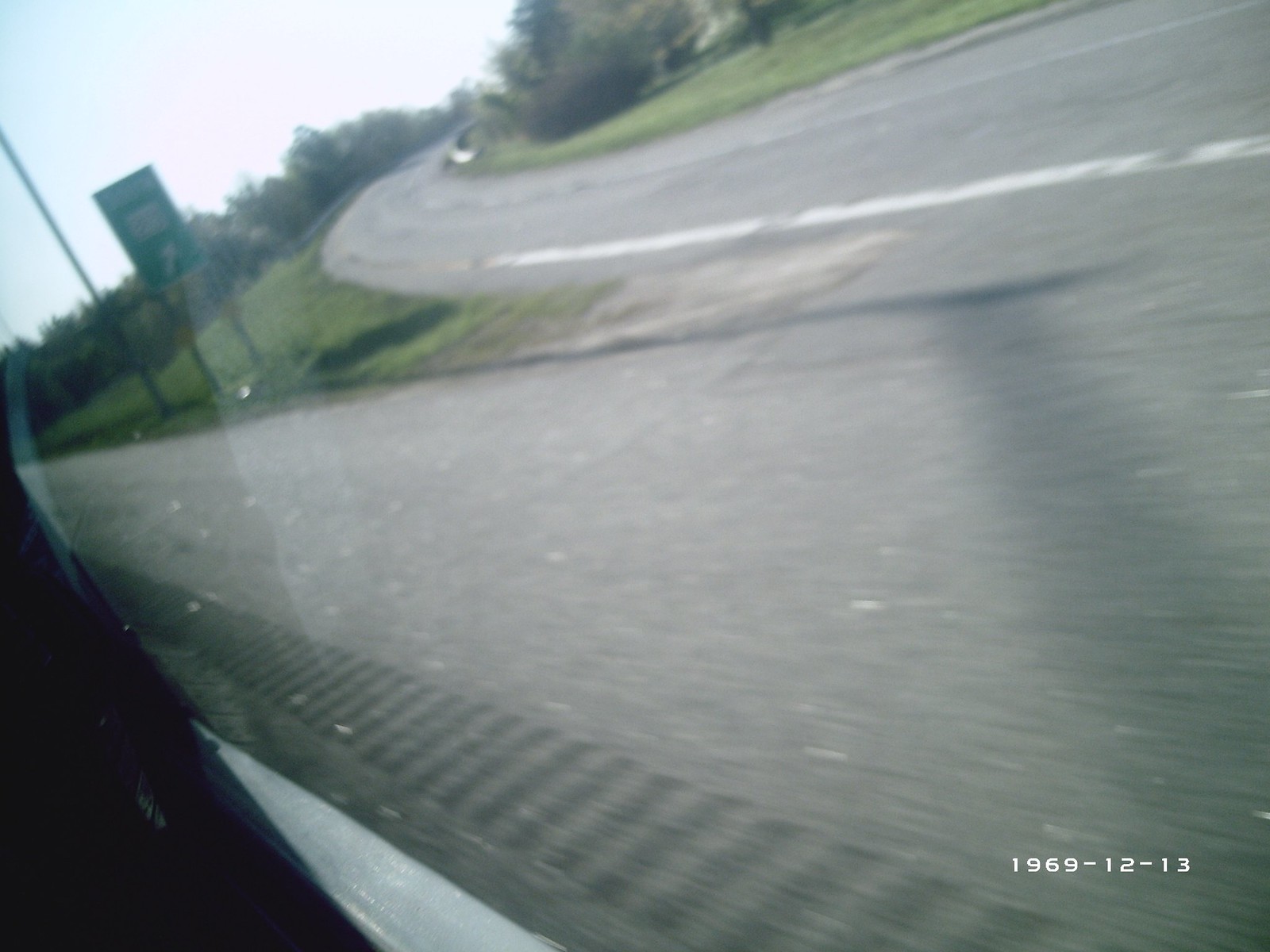The photograph captures a first-person point of view from inside a moving vehicle, possibly from the passenger seat, looking out through the car window. The image is somewhat blurry, which suggests the car is in motion. You can spot the bottom left corner of the vehicle's interior and a slight reflection in the window. The scene outside reveals a highway with a shoulder marked by those tactile bumps designed to wake up motorists drifting off the road. The image also shows a road diverging into an exit on the right. This exit leads off to another direction, curving up and around, with a green road sign sporting a white arrow indicating the exit. While the text on the sign is illegible due to the blur, it likely says "Exit." At the bottom right corner of the image, the date "1969-12-13" is clearly visible. The background scenery includes dark green trees and patches of green grass.